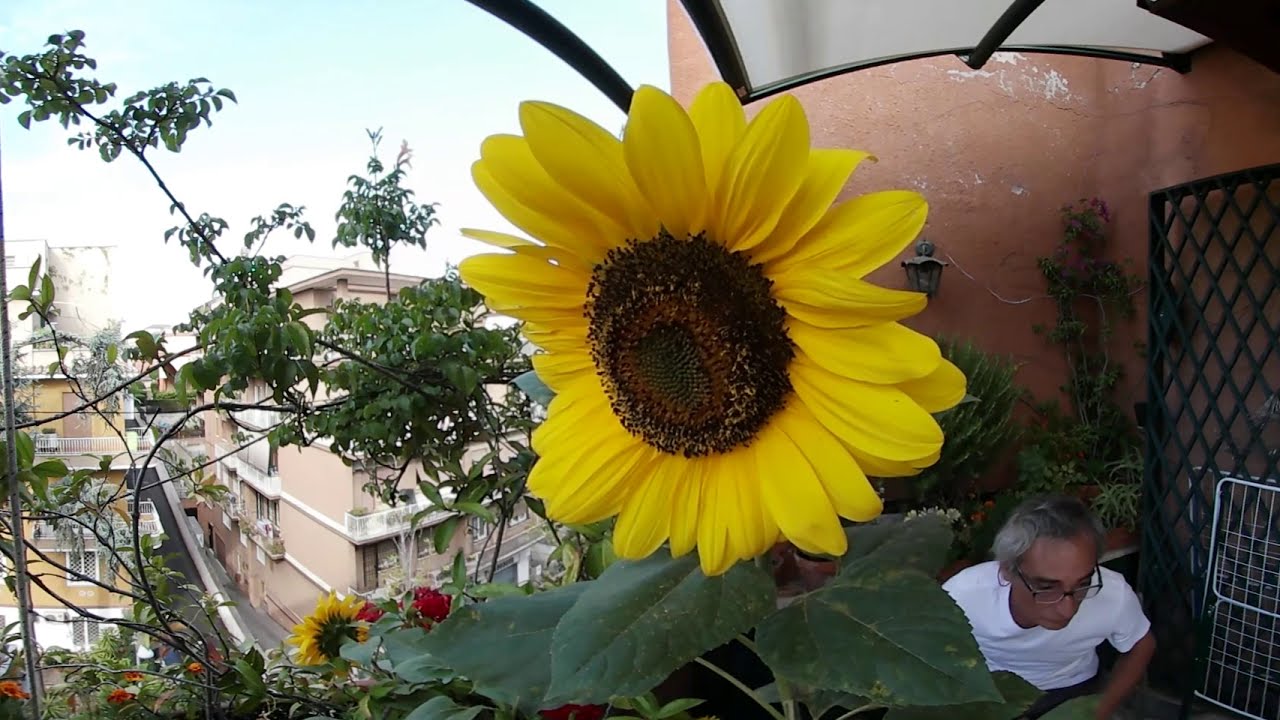In this vibrant outdoor image taken on a clear, beautiful blue day, a high-up balcony garden is captured in full bloom. Central to the composition is a strikingly large, bright yellow sunflower with dark green leaves and a detailed brown center, featuring a dark burnt-yellow ring and tiny budding florets. To the left of the sunflower, red and orange flowers add to the colorful display, creating a lush scene filled with diverse plant life. A man with glasses and gray hair, wearing a white t-shirt, is crouched down in the lower right corner, looking intently outside the frame. The background reveals a reddish clay-colored wall of the porch adorned with a green lattice and a metal fence door. On the left side, urban buildings and a street are visible, indicating that the garden oasis is part of a balcony several stories up.